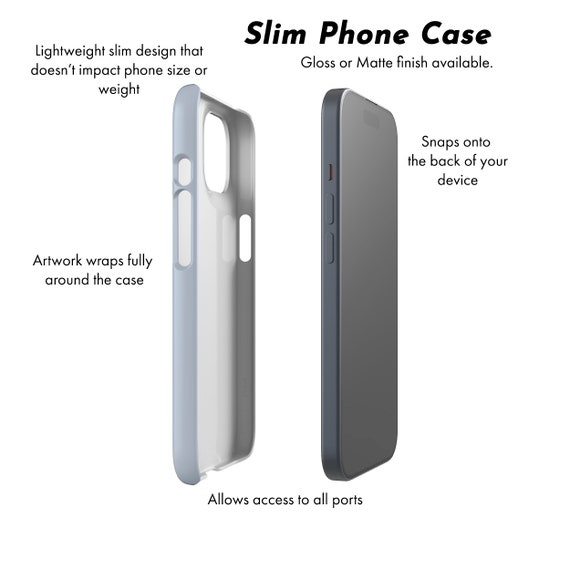The image is a product photo featuring a slim phone case and an iPhone set against a white background. At the top, bold black text reads "Slim Phone Case" with a note below that saying "Gloss or Matte Finish Available." The phone case, displayed on the left, is a sleek white or silvery white color, and the iPhone on the right is a basic gray, with visible volume and silencer buttons but otherwise nondescript. Surrounding the devices, clockwise starting from the top left, are multiple descriptors in black text: "Lightweight slim design that doesn't impact phone size or weight," "Artwork wraps fully around the case" (though the displayed case is plain white), "Allows access to all ports," and "Snaps onto the back of your device." The overall layout resembles a diagram, emphasizing the features and minimalist design of the phone case.